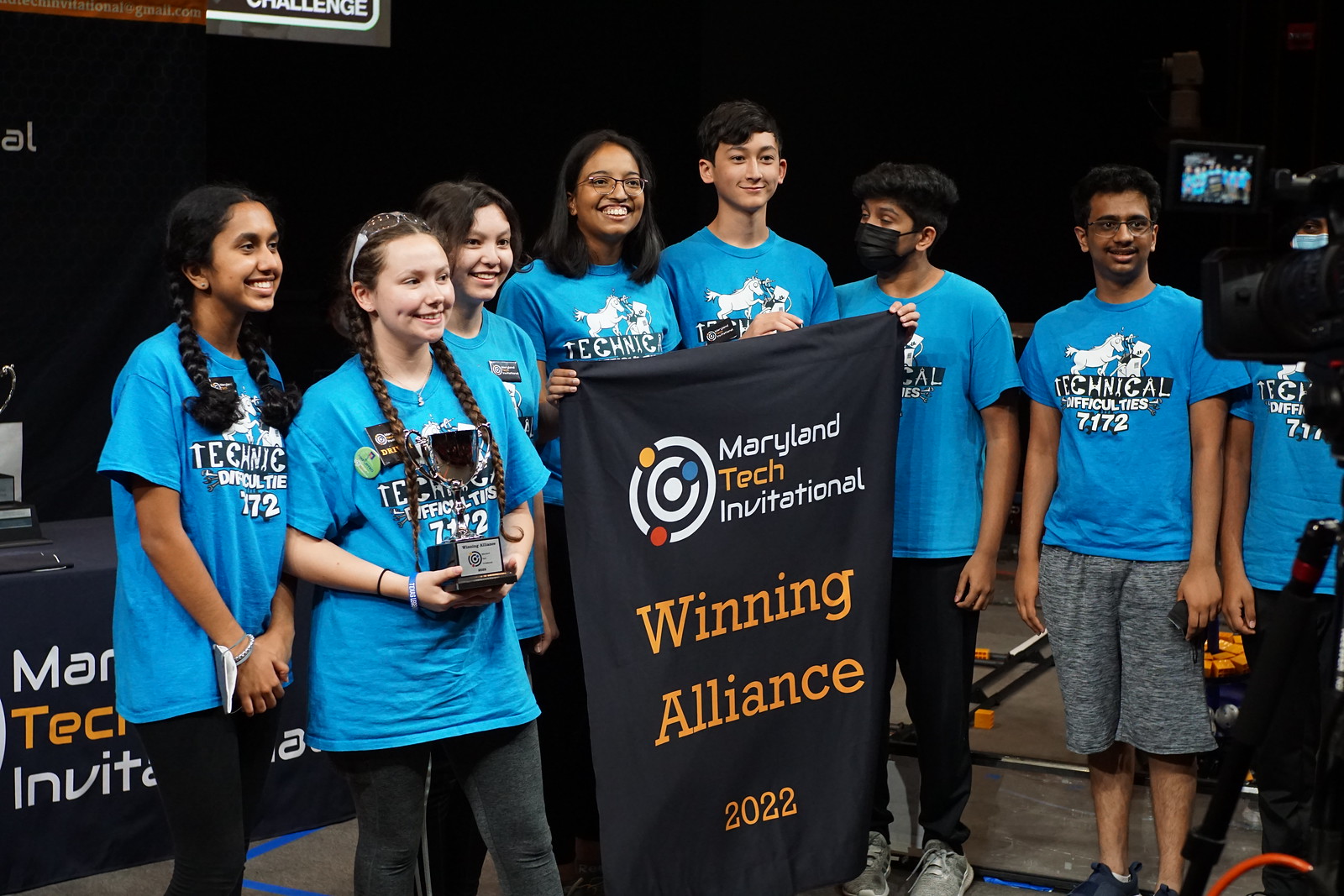The image depicts a group of high school students receiving an award at a scientific competition. They are dressed in identical blue T-shirts featuring a graphic of a horse at a computer and the text "Technical Difficulties 7172." The group, comprised of seven individuals—four girls on the left and three boys on the right—stand against a dark black background. Notably, one girl on the left is holding a trophy with a dark base and a silver placard. Another boy and girl hold up a large black cloth banner that reads "Maryland Tech Invitational Winning Alliance 2022" in gold letters. Among the group, the two girls on the far left have long braided hair, and the sixth person from the left is the only one wearing a mask.